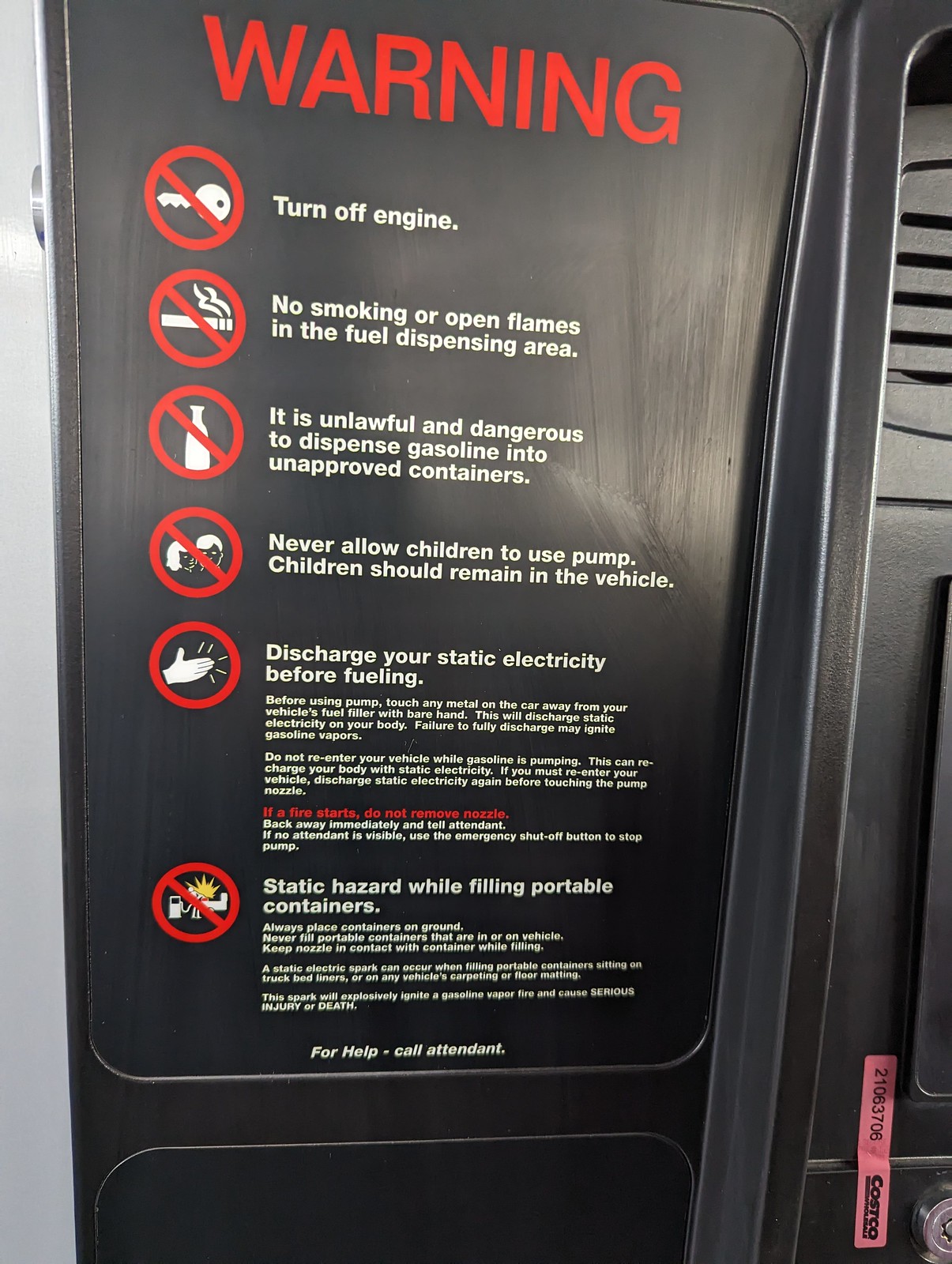The image is a detailed color photograph of a warning sign in portrait orientation, positioned at a gas station beside a partially visible, black fuel dispensing machine. Dominating the center, the sign is black with bold red text at the top reading "WARNING." Below this, there are six warning symbols, each depicted as a white illustration surrounded by a red circle with a diagonal slash through it, indicating prohibition. The first symbol is a white key with the instruction "TURN OFF ENGINE." The second symbol features a lit cigarette, accompanied by the text "NO SMOKING or OPEN FLAMES in the fuel dispensing area." The third depicts a gasoline container and states, "It is unlawful and dangerous to dispense gasoline into unapproved containers." The fourth shows two children with the caution "NEVER ALLOW CHILDREN TO USE PUMP. Children should remain in the vehicle." The fifth illustrates a hand with lines signifying static and advises, "DISCHARGE ALL STATIC ELECTRICITY BEFORE FUELING." Lastly, at the bottom, a fuel pump illustration warns of a "STATIC HAZARD WHILE FILLING PORTABLE CONTAINERS." The sign concludes with instructions stating, "For help call attendant." The detailed symbols and text ensure clear communication of safety precautions to avoid hazards at the fuel dispensing area.